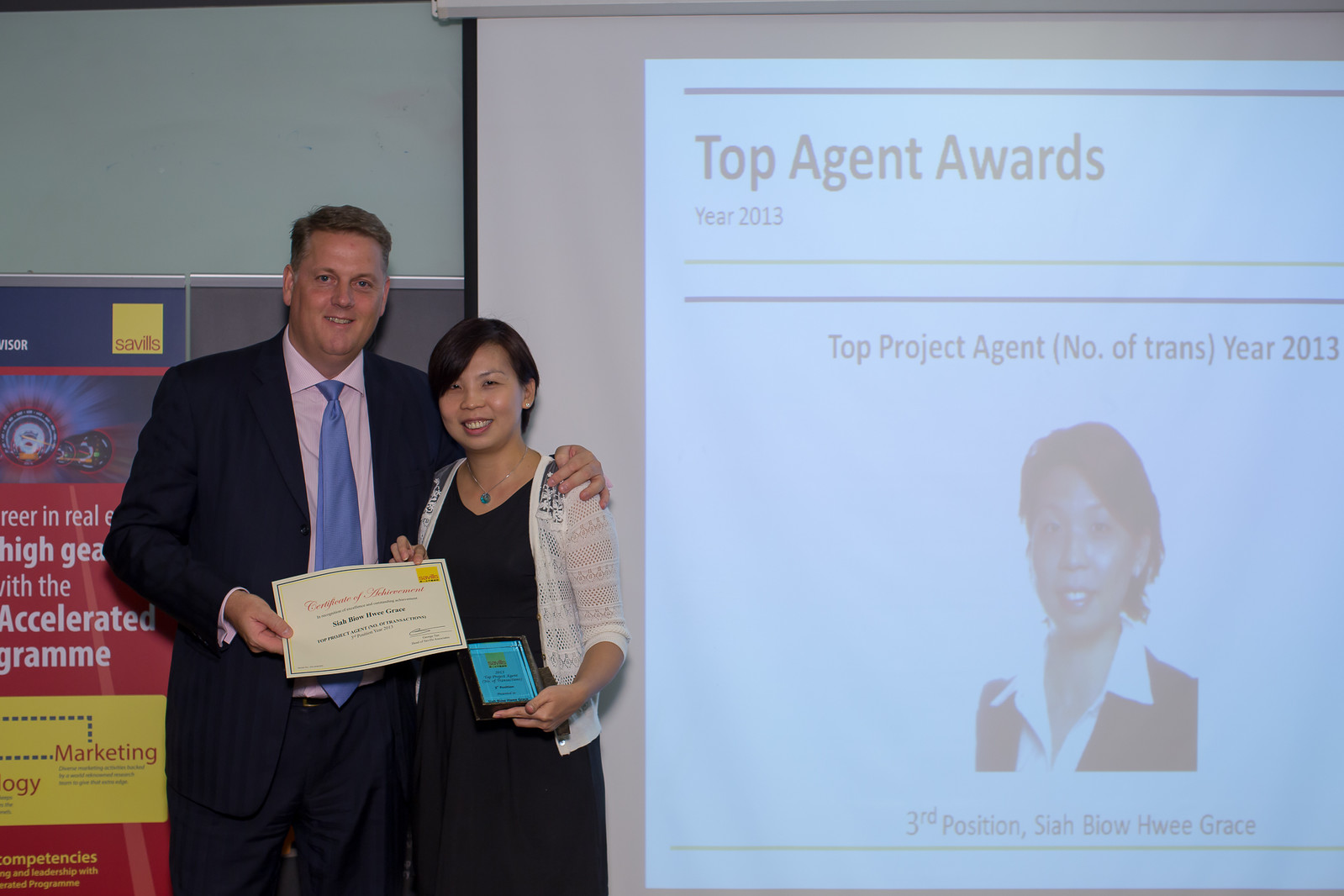In this image, two individuals are prominently positioned in front of a projector screen against a green wall. The man on the left, who is dressed in a navy suit with a pink button-down shirt and a blue tie, stands with his left hand resting on the shoulder of the woman. She has short black hair and is wearing a black dress paired with a white cardigan. They are standing to the left of the projected image on the screen.

The projector screen displays the title "Top Agent Awards, Year 2013," and further down, it reads "Top Project Agent, [Bracket Number of Chance], Year 2013." Below these titles is a faded image of the award recipient, an elegant Asian woman donning a white collared shirt and a black vest. The woman in real life, standing to the left of the screen, is holding a Certificate of Achievement, confirming her recognition as the Top Project Agent for 2013. Her name, Sia Biao Howie Grace, is clearly visible on the certificate. The scene encapsulates the moment of her receiving the award, commemorating her accomplishment.